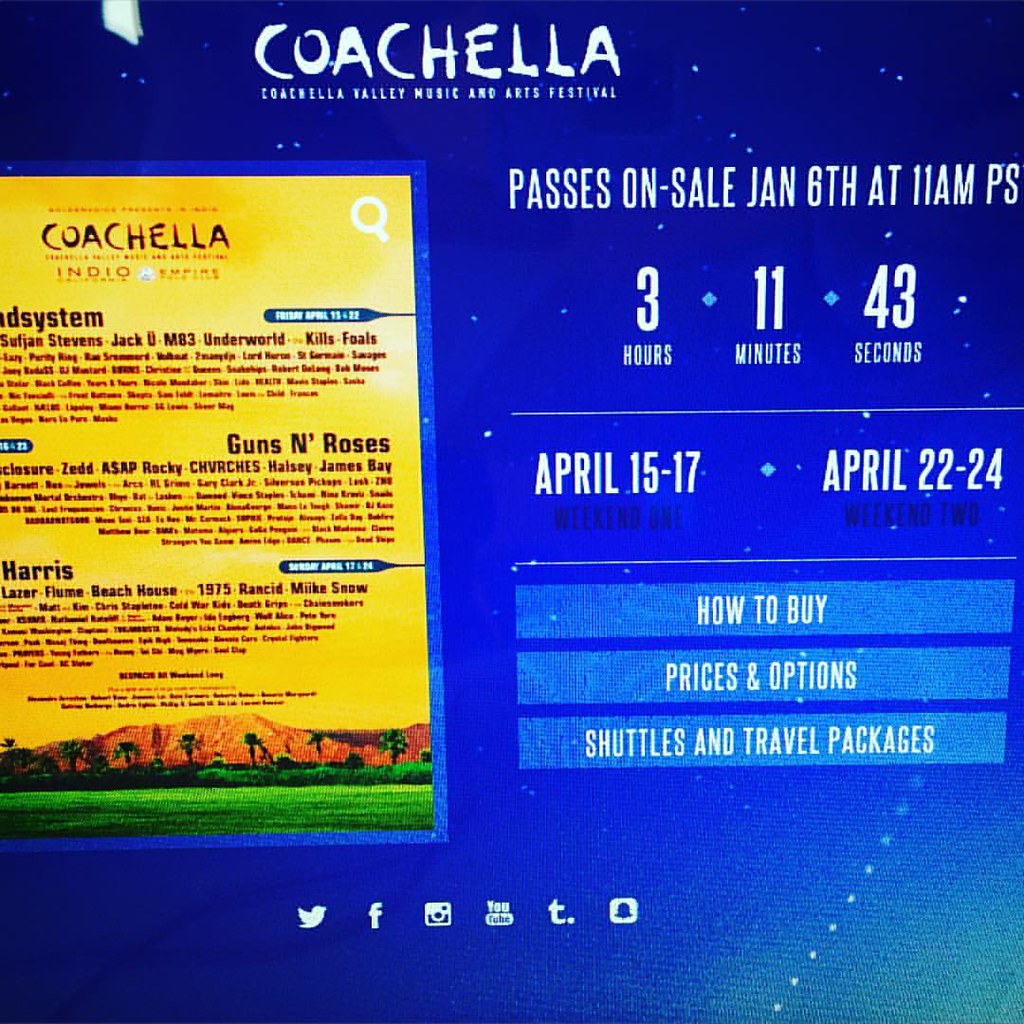The image is a detailed screenshot of a website dedicated to the Coachella Valley Music and Arts Festival. Dominated by a deep blue background reminiscent of a starry night sky, the page prominently features the Coachella logo at the top, styled in white, painted capital letters. Below this, the words "Coachella Valley Music and Arts Festival" are displayed. 

On the left side of the screen, there is a bright yellow flyer showcasing an extensive list of bands performing at the festival, including notable names like Guns N' Roses among approximately 70 to 80 other artists. The flyer also displays imagery of grass and a horizon at its lower edge, organized into three paragraphs of artist names.

At the center-right, the website announces "Passes on sale January 6th at 11 a.m. PST," accompanied by a countdown clock that reads "3 hours, 11 minutes, 43 seconds." The festival dates are marked clearly: April 15th-17th for Weekend 1 and April 22nd-24th for Weekend 2. 

Strategically placed below this information are three interactive buttons labeled "How to Buy," "Prices and Options," and "Shuttle and Travel Packages." Further down, a series of social media icons provide quick access to platforms like Twitter, Facebook, and Instagram. This layout serves as an informative guide for prospective attendees on ticket purchasing and festival details.